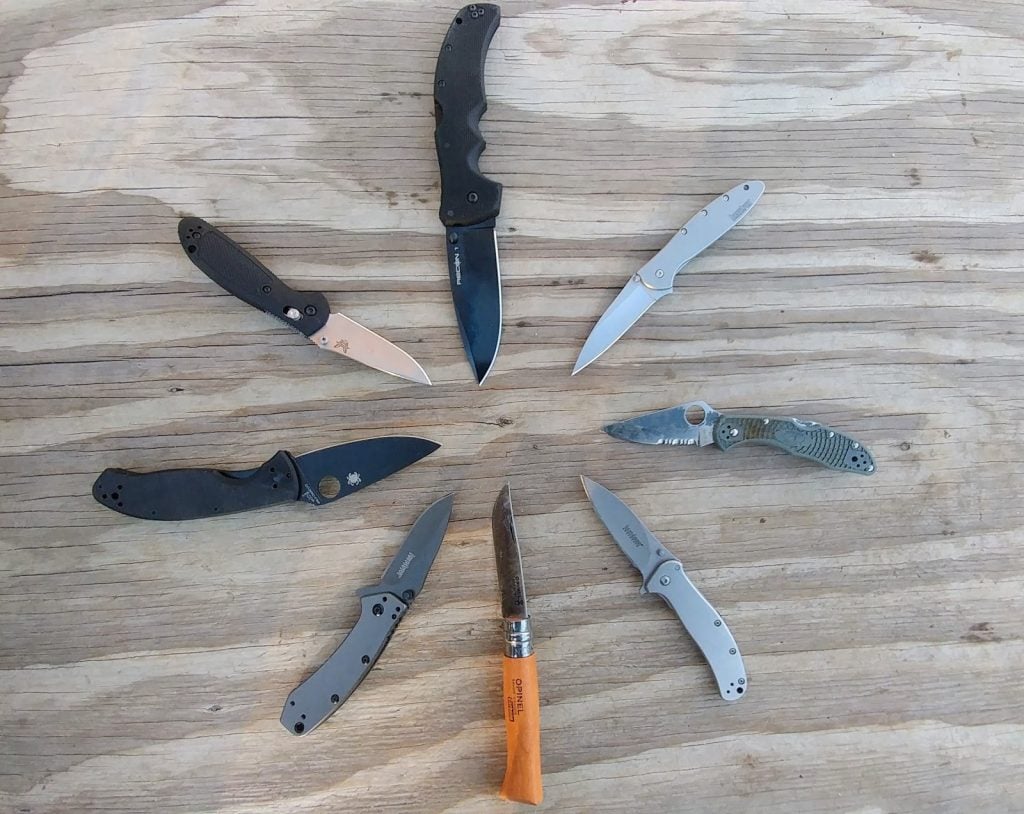The image depicts a top-down view of eight paring knives meticulously arranged in a circular pattern on a grayish-beige wooden surface. All the knife blades are pointed inwards, converging at the center of the circle. Starting from the top center position, akin to the 12 o'clock mark on a clock, and moving clockwise: there is a knife with a black handle, followed by a silver-handled knife, then a metal-handled knife in a darker gray shade, another silver metal handle, a knife with a yellow-golden wooden handle, another knife with a gray metallic handle, and finishing with two black-handled knives at the 7 and 9 o'clock positions. Each knife varies in size and handle design, contributing to the diverse yet harmonious arrangement on the patchy wooden surface.